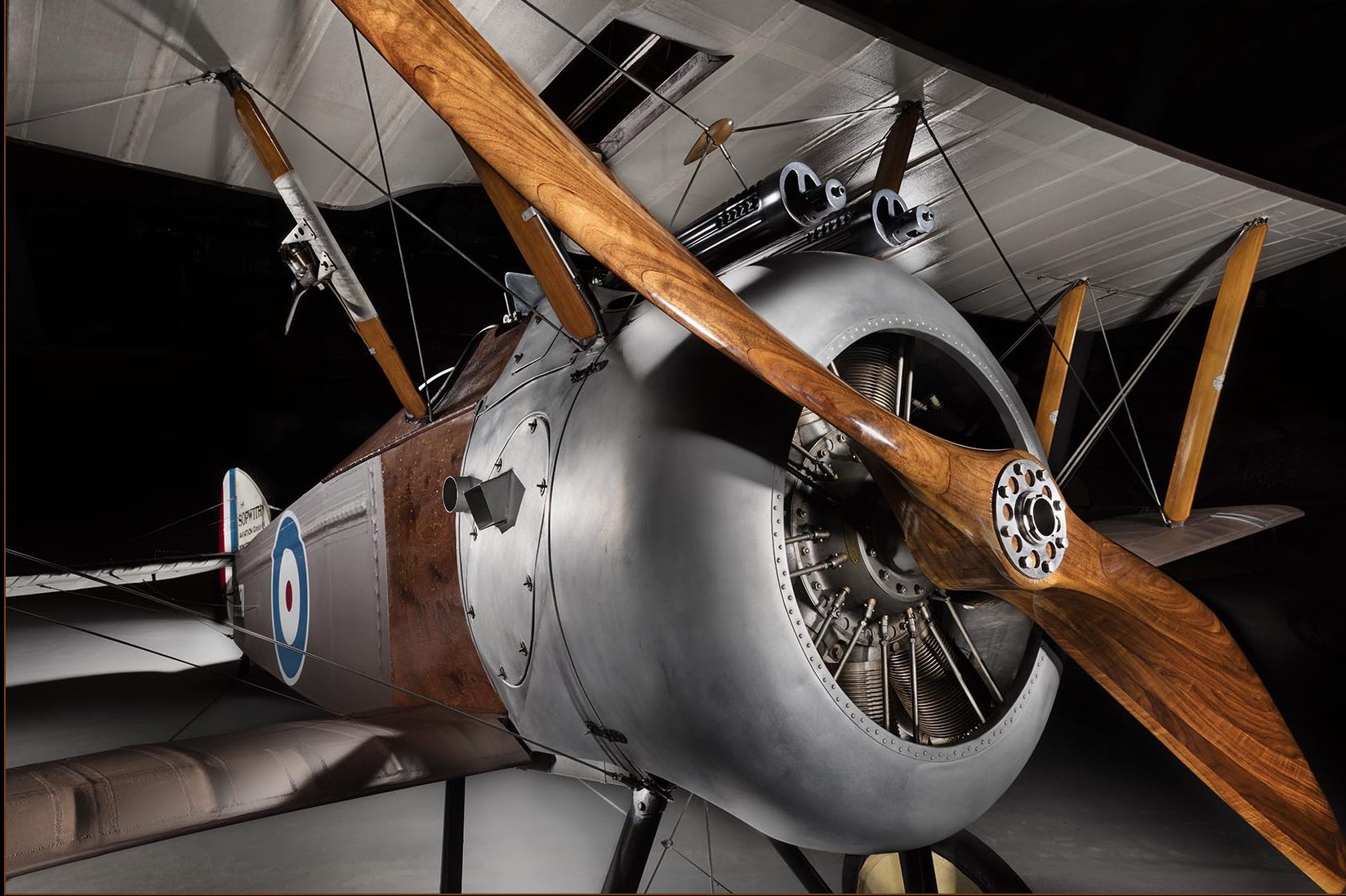This photograph captures a meticulously preserved World War I-era biplane on display in what appears to be a museum, its intricate details illuminated against a black backdrop. The aircraft features a distinctive dual-wing design, with one wing positioned above the other and supported by wooden struts both at the edges and the body of the plane. The bottom of the upper wing is white, complementing the grayish hue of the plane’s front section. Prominently mounted on the nose is a finely crafted wooden propeller, capped with a metal piece. Just behind the propeller, a radial engine with a grayish tinge is clearly visible, alongside two machine guns affixed atop the engine casing. Additional features include two exhaust pipes on the right side— one square-shaped and the other round.

An emblem adorns the tail of the aircraft, displaying a red dot encased within a white circle, followed by a larger bluish circle, and encircled by a solid white line. The tail also bears unreadable lettering, except for an initial 'S'. A prominent red, white, and blue stripe can be seen on the very back of the plane. Moreover, the floor beneath the plane reflects the light shining from off-camera, enhancing the metallic and wooden accents of the biplane. This rich detail coupled with the muted background and precise lighting draws significant attention to the historic and structural nuances of this early 20th-century aircraft.